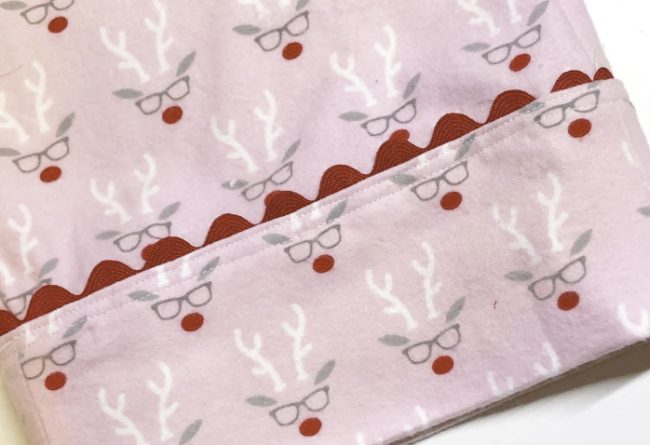This image showcases a piece of light pink fabric, most likely the long sleeve of a pajama top, against a white backdrop. The intricate design on the fabric features a whimsical pattern of deer faces. Each face is composed of white antlers and gray eyebrows above dark gray eyeglasses, with red dots positioned below to depict noses. The faces are arranged in neat rows, creating a playful and consistent motif throughout the fabric. The bottom hem of the sleeve is adorned with a distinctive red, wavy rickrack trim, made from a different material, which adds a charming, tactile contrast and matches the red noses in the pattern. The overall detail and alignment suggest a carefully designed and cozy piece of sleepwear.